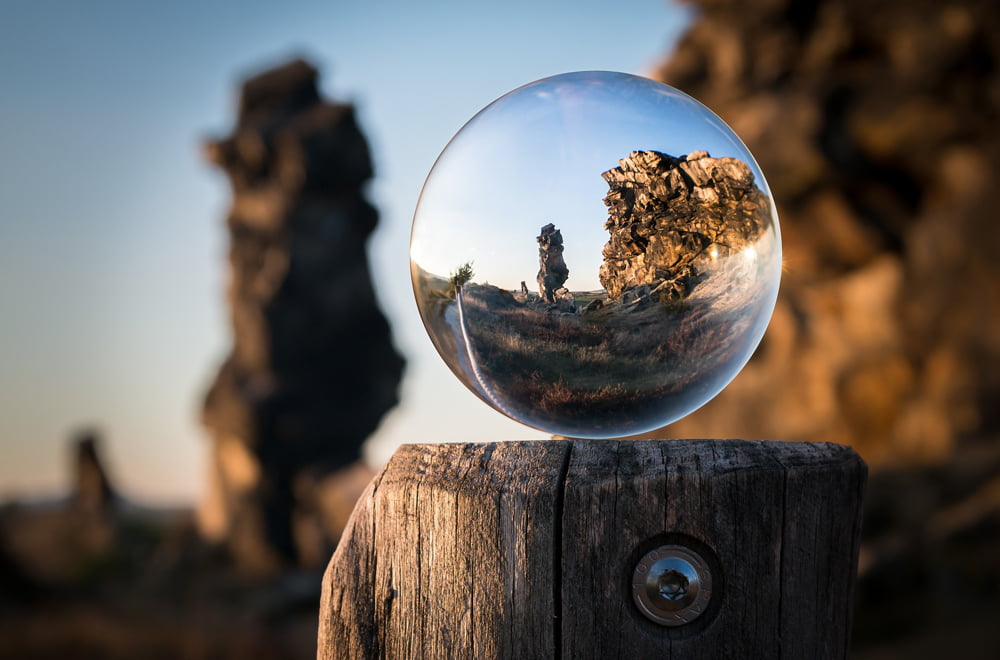In this captivating photograph, a delicate glass orb rests atop a wooden post, which is centrally positioned in the foreground on the right side of the frame, occupying approximately 25% of the image’s height. The wooden post, marked by a visible silver bolt, serves as a sturdy pedestal for the orb. The image's focal point, the glass orb, acts as a transparent lens, bringing clarity to the otherwise blurred background. Through the orb, you can distinctly see stone outcroppings: a large formation to the right and two smaller ones to the left. The crisp, blue sky frames the scene beautifully, contrasting with the natural brown tones of the post and the intricate details captured within the glass sphere. The overall effect is an enchanting blend of sharp and soft focus, making the glass orb a mesmerizing centerpiece that draws the viewer's eye.